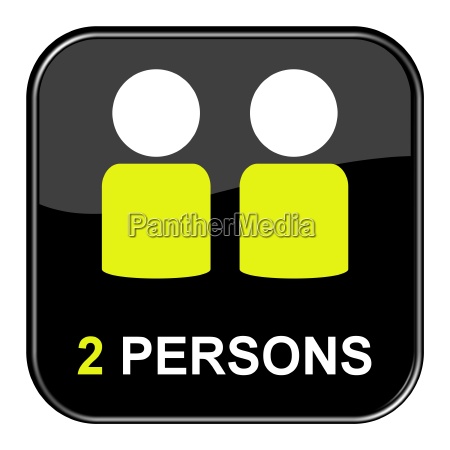The image features a digitally created clip art positioned in the center of a solid white background. At the center of the image, there is a black square with rounded edges, inside which two stylized figures representing people are depicted. Each figure consists of a white circle for the head and a yellow, block-shaped rectangle for the body. The background within the square is multicolored, incorporating shades of white, gray, black, white, and lime green. The top of the square bears a watermark reading "Panther Media," while the bottom text reads "Two Persons," with the word "Persons" in white and the number "2" in yellow. The design is cleanly laid out, emphasizing the theme of seating or occupancy for two individuals.